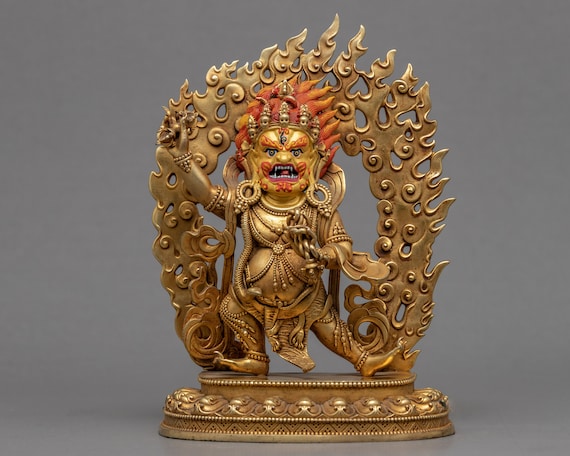The image showcases a detailed statue that appears to be significant in Hindu or Buddhist mythology, potentially of a deity or demon. The statue has a fierce, wide human-like face with sharp pointy teeth and a scowling expression. Its eyebrows and hair are depicted as flames, containing small faces or skulls. It dons a headdress reminiscent of flames and features jewelry that partially covers its exposed stomach and chest. The being is adorned with large circular earrings, a crown-like headpiece, and jewelry around its legs. A snake drapes around its neck, adding to its dramatic appearance.

One hand of the statue is raised, holding an unidentifiable object, while the other hand extends, possibly holding chains. The figure is poised with one leg extended out and stands within a circular ring of fire. The statue, made of what appears to be brass or gold, rests on an oval-shaped base, against a neutral gray background. This richly detailed representation likely holds cultural and religious significance in East or Southeast Asian traditions.